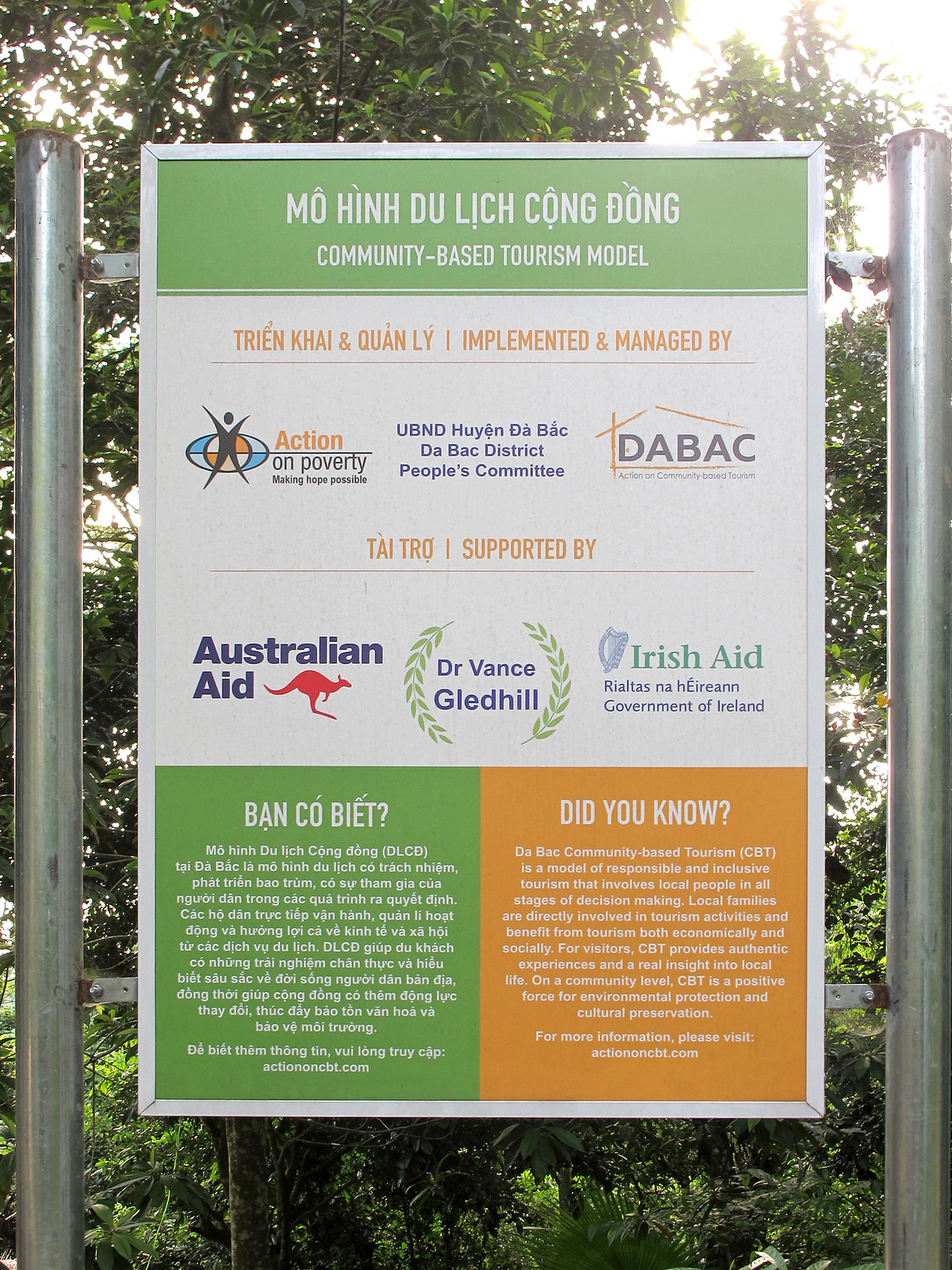This outdoor photograph, taken on a sunny but not overly bright day, showcases a silver post with a bit of rust, holding a prominent advertisement sign. The backdrop features lush green trees and a clear sky, particularly bright in the upper right-hand corner. The sign, centered between two supportive poles, stands out with its green, white, and orange colors. It announces the "Mo Hong Dong, Lich Kong Dong Community-Based Tourism Model" and includes an array of details in both English and another language. Clearly stating "Implemented and Managed by Action on Poverty," it lists contributors such as Tran, Cal, and Kwan Lee. The advertisement features logos and mentions various supporters, including UBND, the People's Committee, D-A-B-A-C with a symbol resembling a house, Australian Aid with a kangaroo logo, as well as Dr. Vince Glynn-Hill, and Irish Aid, depicted with wheat symbols. At the bottom, the sign highlights in orange text: "Did You Know," along with a mention of the website Action on CBT.com, emphasizing the model's aim to involve local people in all stages of responsible and inclusive tourism decision-making.